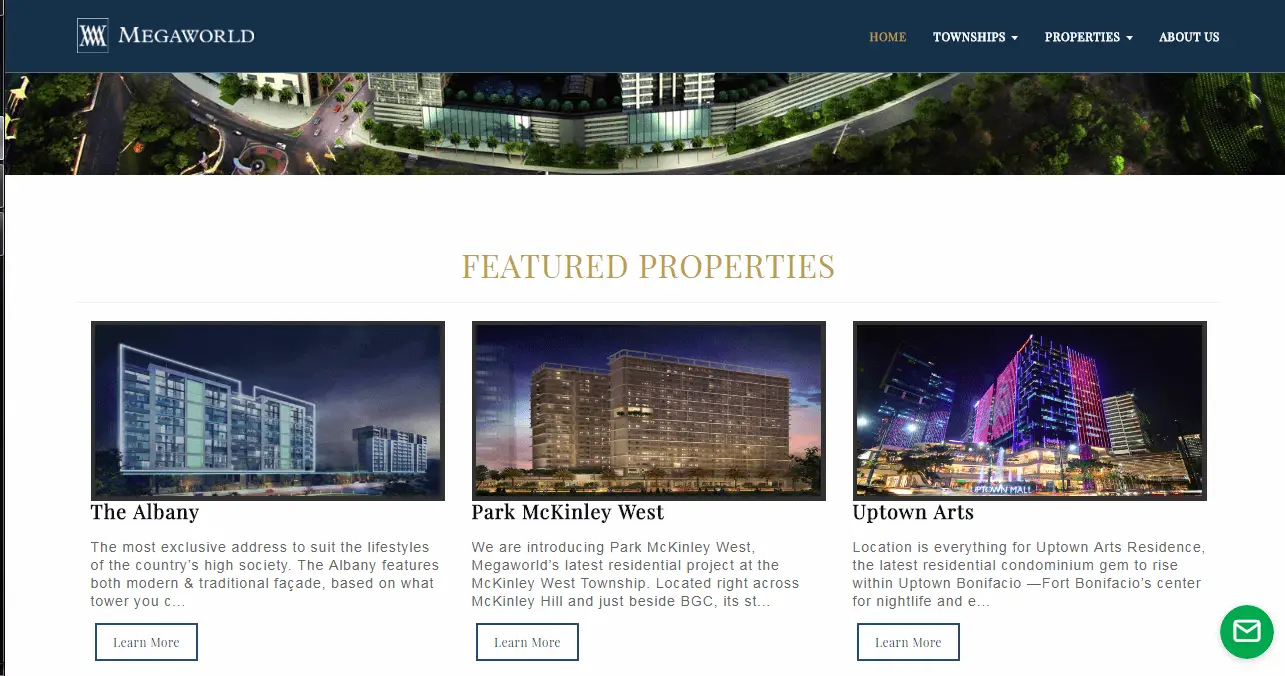The top section displays a navy blue background header. Towards the right, there are several menu options. The first option, "HOME", is written in capital letters with a Times New Roman font, styled in a taupe or beige color. The next option, "TOWNSHIPS", is in white with a downward arrowhead indicating a drop-down menu. Following that, "PROPERTIES" is showcased, also with an arrowhead pointing to the right, suggesting another drop-down menu. The last option is "ABOUT US".

On the left side of this header, in capital letters, "MEGA WORLD" is written in white, positioned next to a logo consisting of an overlapping "M" and "W". This logo features a white border.

Below this header, there is a long banner displaying the lower part of a city building. Underneath the banner, the background transitions to white. In the middle, golden capitalized letters spell out "FEATURED PROPERTIES". 

Following this text, images of three different properties are presented. The first property, "The Albany," features three blue, square-shaped buildings set against a night sky. The second property, "Park McKinley West," shows two golden-colored buildings with a backdrop of a pink and purple sunset. The third property, "Uptown Arts," highlights a square building from a bottom-up view, adorned with pink and purple panels.

At the bottom of each property listing, there is a rectangular icon with a black border containing the text "LEARN MORE."